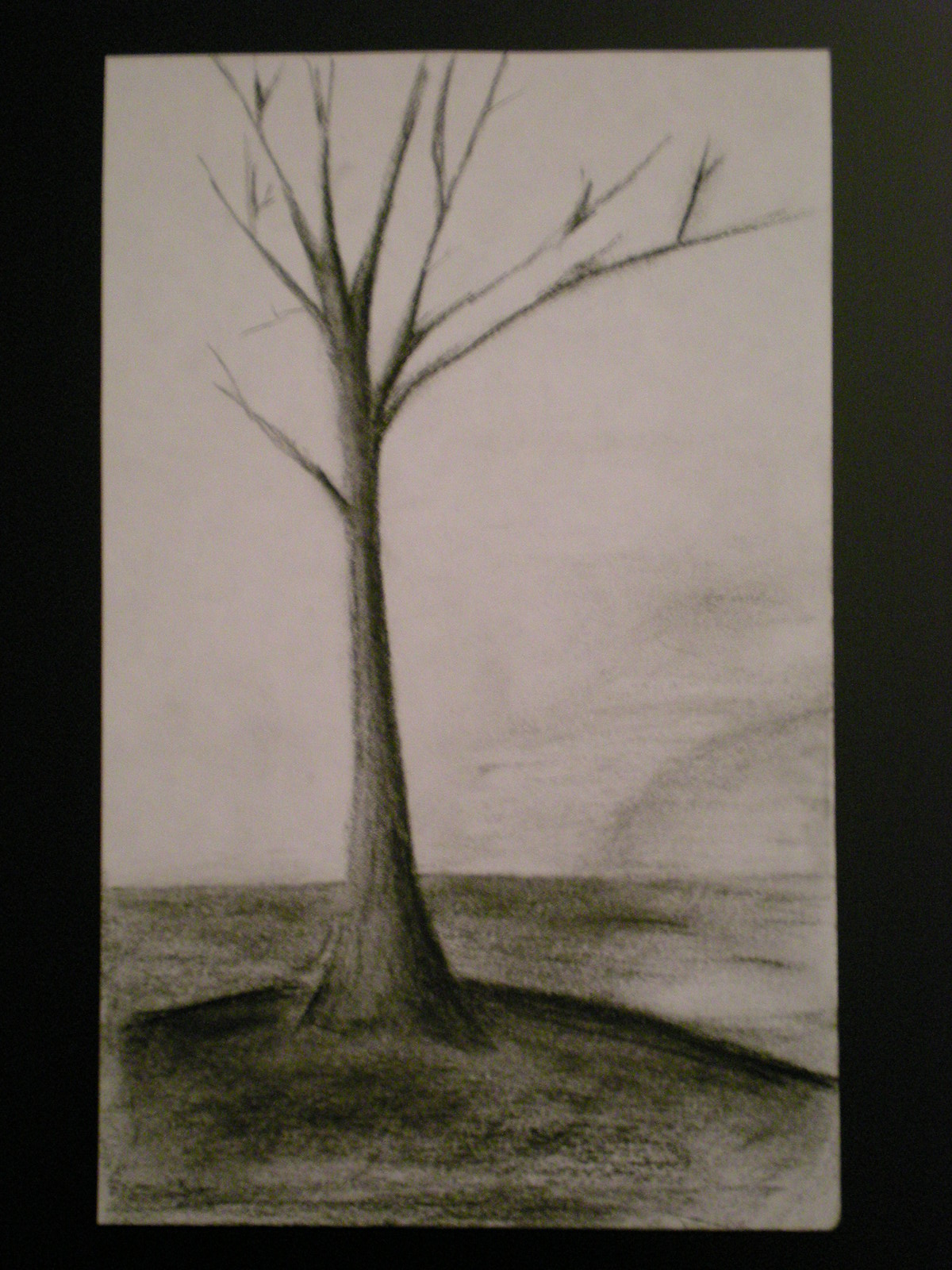This is a detailed photograph of a drawing, prominently featured against a completely black background which may either be a wall or a table surface. The drawing is on a piece of paper that appears to be medium to light gray, oriented vertically. The artist has skillfully utilized pencil, charcoal, or graphite to create a finely rendered landscape.

The ground is beautifully depicted with a wide range of shades, from very bold blacks to the lightest of grays, showcasing the artist's adept use of gradients. A single, narrow-trunked tree grows out of a delicately shaded mound. The tree is characterized by its spindly form, minimal branches, and lack of leaves, adding a stark but elegant focus to the composition.

In the background, the horizon is subtly indicated with soft shading, adding depth to the scene. The sky above is rendered with very light shading, punctuated by a few delicate clouds on the right side, giving a sense of stillness and tranquility to the overall image. This detailed and expressive drawing captures the serene beauty of a solitary tree in a minimalist landscape.